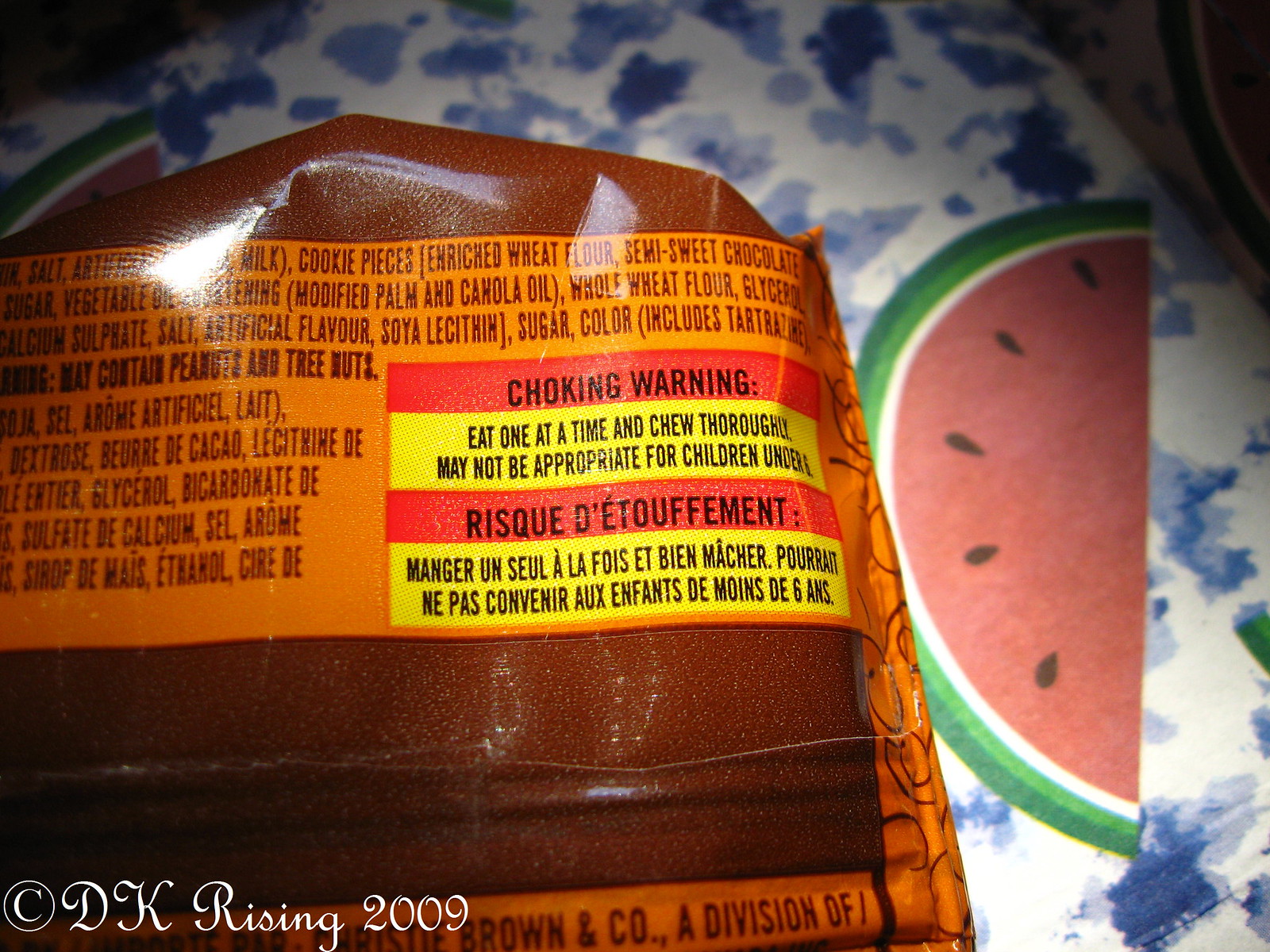This image depicts the back of a brown food package with an orange label and trim, lying on a blue and white tablecloth adorned with watermelon wedges. The text on the packaging is in both English and French, including a clear choking warning that reads: "Eat one at a time and chew thoroughly. May not be appropriate for children under six." A copyright notice in white text on the lower left corner states "© DK Rising 2009." Alongside the warning, partial ingredients are visible, listing components like wheat flour, semi-sweet chocolate, modified palm and canola oil, whole wheat flour, glycerin, sulfate, salt, artificial flavor, soy lecithin, and sugar, indicating the possible presence of cookies. The watermelons on the tablecloth are detailed with dark green rinds, light green margins, white, and pink flesh, with black seeds scattered throughout. The package's text appears primarily in black and is complemented by warnings and other details in red and yellow.